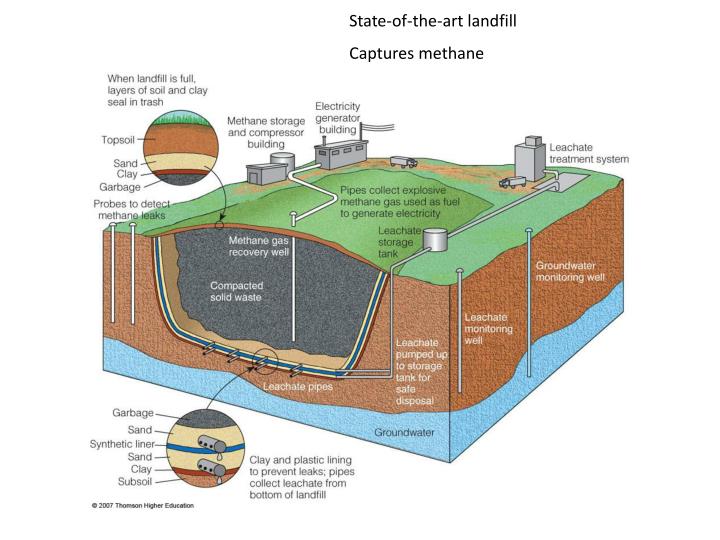This detailed infographic, possibly from a 2007 textbook by Thompson Higher Education, illustrates the process of methane capture in a state-of-the-art landfill. The top of the image features the text, "state-of-the-art landfill captures methane." The diagram shows a cross-section of a landfill with various components and processes involved in methane capture and environmental safety.

The landfill is sealed with layers of topsoil, sand, and clay to contain the trash. Probes are installed to detect methane leaks. Methane gas is collected through a series of pipes and stored in a methane storage and compressor building. The methane is then used as fuel to generate electricity in an electricity generator building. Additionally, the diagram depicts a leachate storage tank and a sophisticated treatment system to collect and manage leachate from the bottom of the landfill. Monitoring wells are in place to ensure groundwater safety, and clay and plastic liners prevent leaks. The color coding in the image includes green for the grass layer, brown for dirt, silver for pipes, and blue for groundwater, providing a clear and organized visual of the entire methane capture process.